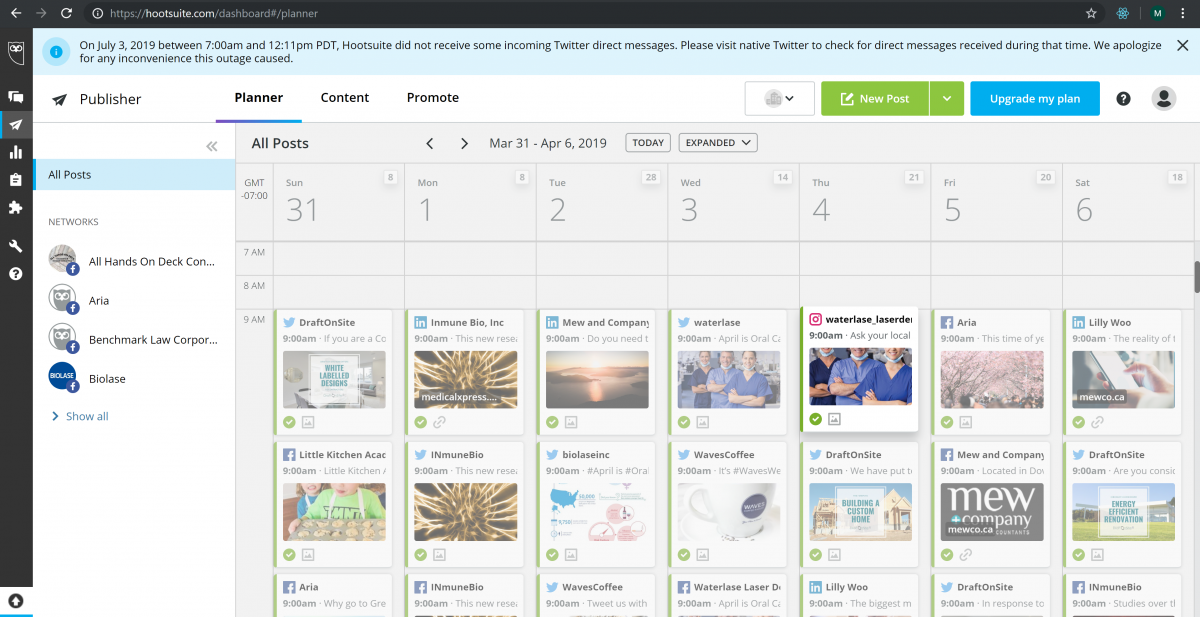The image captures a computer screen displaying the Hootsuite dashboard. At the top, a black border frames the screen with the browser URL bar visible, indicating a secure HTTPS website. Below the URL bar is a notable announcement encased in a blue border, stating: "On July 3, 2019, between 7 a.m. and 11:59 p.m. PDT, HootSuite did not receive some incoming Twitter direct messages. Please visit native Twitter to check for direct messages received during that time. We apologize for any inconvenience this outage caused."

On the left side of the screen, within a black-bordered sidebar, multiple icons are visible, including a wrench, a question mark, three horizontal bars, and an envelope, likely representing various functionalities and settings. Adjacent to this sidebar, a section titled "All Posts" is highlighted in blue, indicating it's the currently active tab.

To the right, against a white background, a calendar interface is displayed. The calendar is labeled "March 31 through April 6, 2019," indicating the date range. The "Planner" tab is highlighted, showcasing a weekly view. The days of the week are organized into columns, each containing various images and entries, suggesting a schedule of planned social media posts.